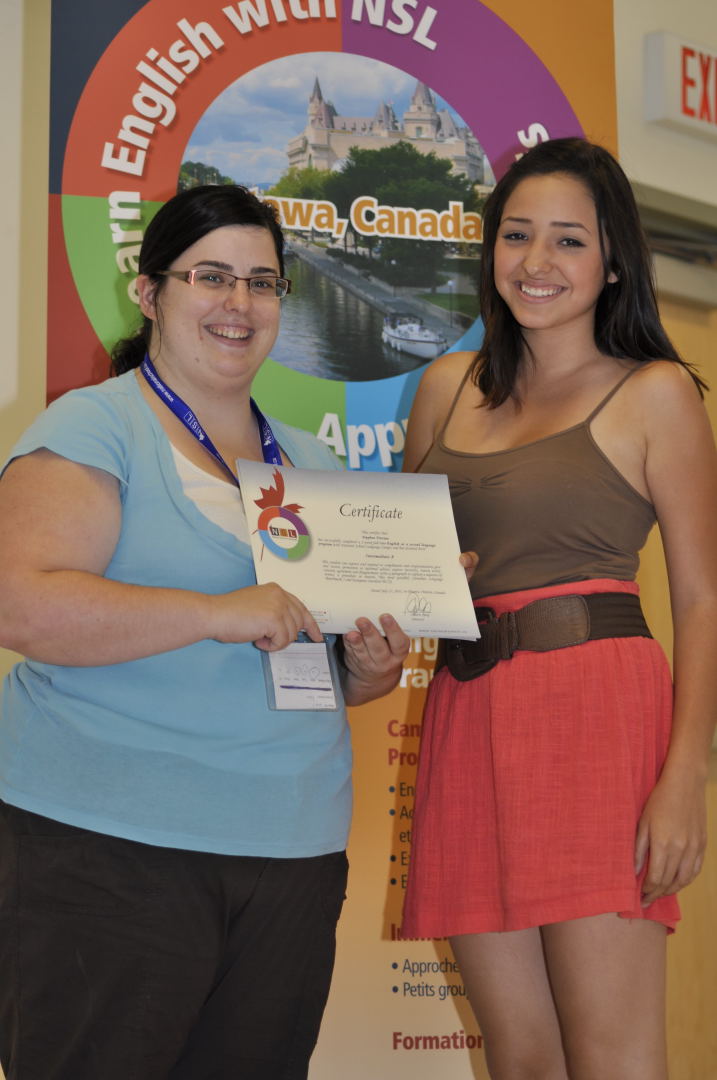The photograph features two women, visible from the knees upwards, standing in front of a banner that reads "Ottawa, Canada" and includes other unreadable text and an image. The woman on the left, facing the camera with her body angled to the left, has pink metallic glasses and wears black pants, a short-sleeved blue shirt over a white undershirt, and a blue lanyard with white text ending in a clear plastic badge holder containing a white piece of paper. She is holding a blue piece of paper that reads "Certificate" in black text. Her black hair frames a smiling face. On the right, a taller woman, also smiling, with olive skin and long dark hair, wears a short orange skirt, a brown fabric belt, and a thin-strapped brown sleeveless tank top. Both women are collectively holding the certificate in the photo.